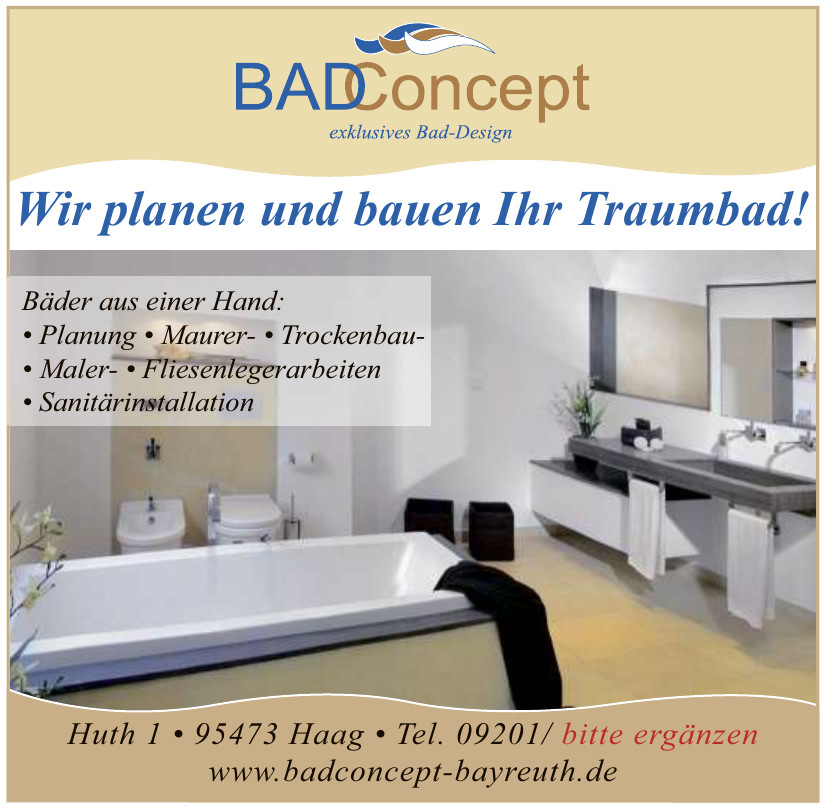The image is an intricately designed advertisement for a company called Bad Concept, and it appears to showcase a luxurious bathroom. At the top of the ad, there is a tan background with a light brown border surrounding the entire image. Centered within the title area, the company name "BAD CONCEPT" is prominently displayed, with "BAD" in bold blue capital letters and "CONCEPT" in brown. The overlapping of the D and C adds a stylish touch. Below the name, italicized text in blue and brown reads "EXCLUSIVE BAD DESIGN," accompanied by a tricolored logo (blue, brown, and white) above the company name.

The central part of the advertisement features a detailed photograph of the bathroom. The bathroom boasts a distinct European style, notably different from typical American designs. Key features include a white square bathtub in the foreground with a black garment draped over its edge, a bidet, and a toilet. On the right, there is a double-sink setup with dual faucets and a mirror above it. Towels hang neatly from rods below the sinks, and the presence of flowers adds a touch of elegance to the space. The bathroom walls are white, and the floor is covered in tan-colored tiles.

In the middle of the image, there is a white box with blue text that reads, "Wir planen und bauen er Trombad!" This appears to be a German phrase related to planning and installing the bathroom. At the bottom of the ad, the contact information is provided in red text, listing the address "Huth 1-95473 Bayreuth" with a telephone number, and the website "www.badconcept-bayreuth.de." The overall design and details of the bathroom along with the company's branding elements indicate a high level of sophistication and attention to detail.